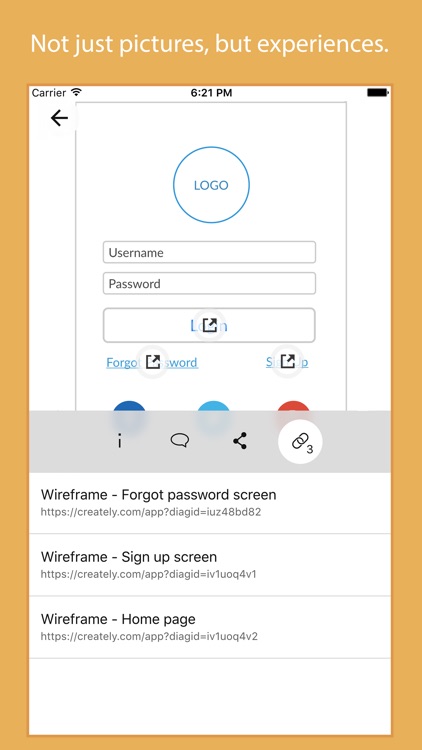The image depicts a cell phone screen with a dynamic user interface theme. The background at the top is a gradient of orangish-yellow, adorned with a white inscription that reads, "Not just pictures but experiences." Below this, the background transitions to white. 

The status bar displays typical elements: the time reads 6:21 p.m., the carrier name is simply noted as "Carrier," and a fully charged black battery icon is also visible. Centered under the status bar, there is a brand logo highlighted in blue, encircled by a blue ring. 

Beneath the logo, there are fields labeled "Username" and "Password" for user credentials. Adjacent to these fields, an upload button is present.

In the middle section, a gray rectangular strip houses four clickable icons: an eye, a speech bubble, a sideways "V," and a link icon labeled with the number "3."

The lower portion of the screen contains navigation options in the format of wireframe labels: 
1. "Wireframe - Forgot Password Screen"
2. "Wireframe - Sign Up Screen"
3. "Wireframe - Home Page"

The very bottom of the screen features an entirely blank white rectangular area, which appears to be unutilized space.